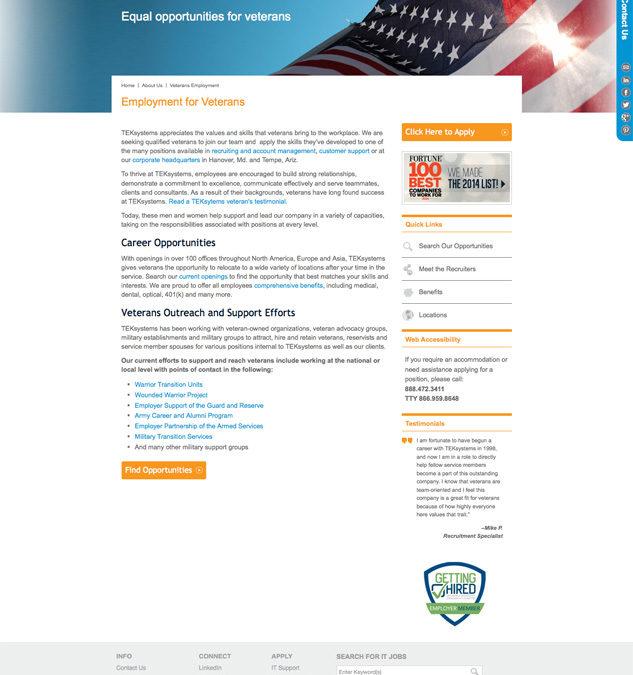This image is a screenshot of a low-resolution, somewhat archaic website focused on veteran employment opportunities. 

At the top, there is a banner featuring a two-toned image: the left side is blue, and the right side displays a partial view of an American flag from a bottom-up angle. The top-left corner of the banner contains white text that reads “Equal Opportunities for Veterans.” A vertical bar on the right side of the banner states “Contact Us” in text displayed vertically, accompanied by various social media icons.

The main content section is organized under several headings. The first line reads “Home,” “About Us,” and potentially “Veterans Employment” (the latter being unclear). Following that, in orange text, it states “Employment for Veterans.” Beneath this heading, the text is mostly illegible due to low resolution.

A dark blue heading labeled “Career Opportunities” follows, accompanied by additional text and light blue hyperlinks embedded within the content. Another dark blue heading, “Veterans Outreach and Support Efforts,” follows. There is supplementary text under this heading, which includes bullet points in medium blue text.

Towards the bottom of the page, there is an orange button labeled “Find Opportunities.” Adjacent to this, on the right-hand side of the page, there is a sidebar containing a clickable item that says “Click Here to Apply.” Beneath it, the text proclaims that the site is listed among the "Fortune 100 Best Companies to Work For," possibly mentioning their place on the 2014 list.

Further down the sidebar, sections labeled “Quick Links,” containing “Search Our Opportunities,” “Meet the Recruiters,” “Benefits,” and “Locations” are listed. This is succeeded by a section dedicated to web accessibility, prefixed by a mention of necessary accommodations (text is not fully legible).

Next, there is a section titled “Testimonials,” which appears to include a pull quote from an individual. 

At the very bottom right, there is a seal that reads “Getting Hired,” with “Getting” in green and “Hired” in blue, incorporated into the design of a blue-outlined shield with a green banner.

Lastly, a gray box at the bottom of the page contains a site map or various links including “Info,” “Connect,” “Apply,” and “Search for IT Jobs.”